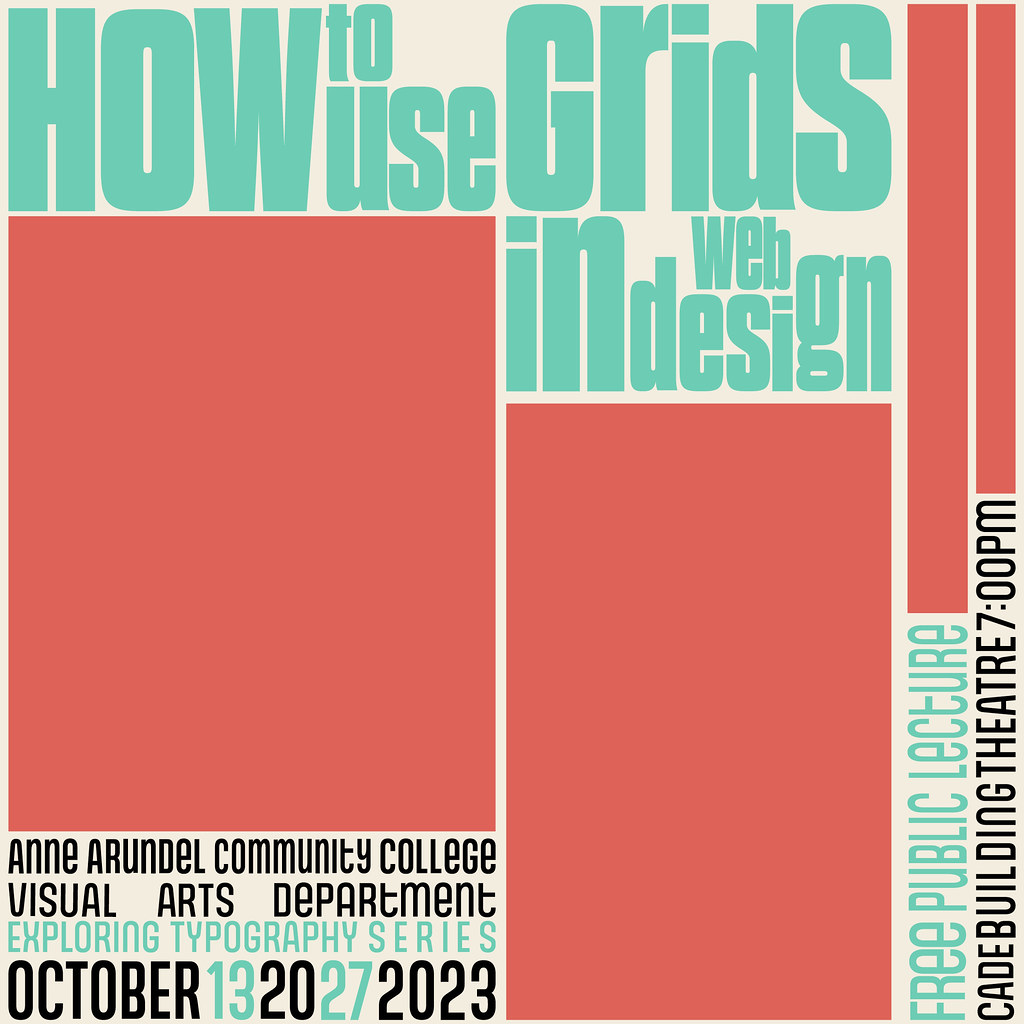The image is a visually structured advertisement for an event, featuring a light blue script at the top that reads, "How to Use Grids in Web Design." To the right of this title, there are four vertically placed rectangles of varying sizes. Directly beneath the two rectangles on the right, it says "Free Public Lecture" in light blue letters, with "Cade Building Theater, 7 p.m." in black letters beside it. On the bottom left, in black script, it reads "Ann Arundel Community College Visual Arts Department," followed by "Exploring Typography Series" in light blue script. Below this, the dates "October 13," "20," and "27" are listed with "13" and "27" in light blue script, and "October" and "2023" in black script. The background of the image has a cream color, effectively highlighting the various textual and graphical elements.